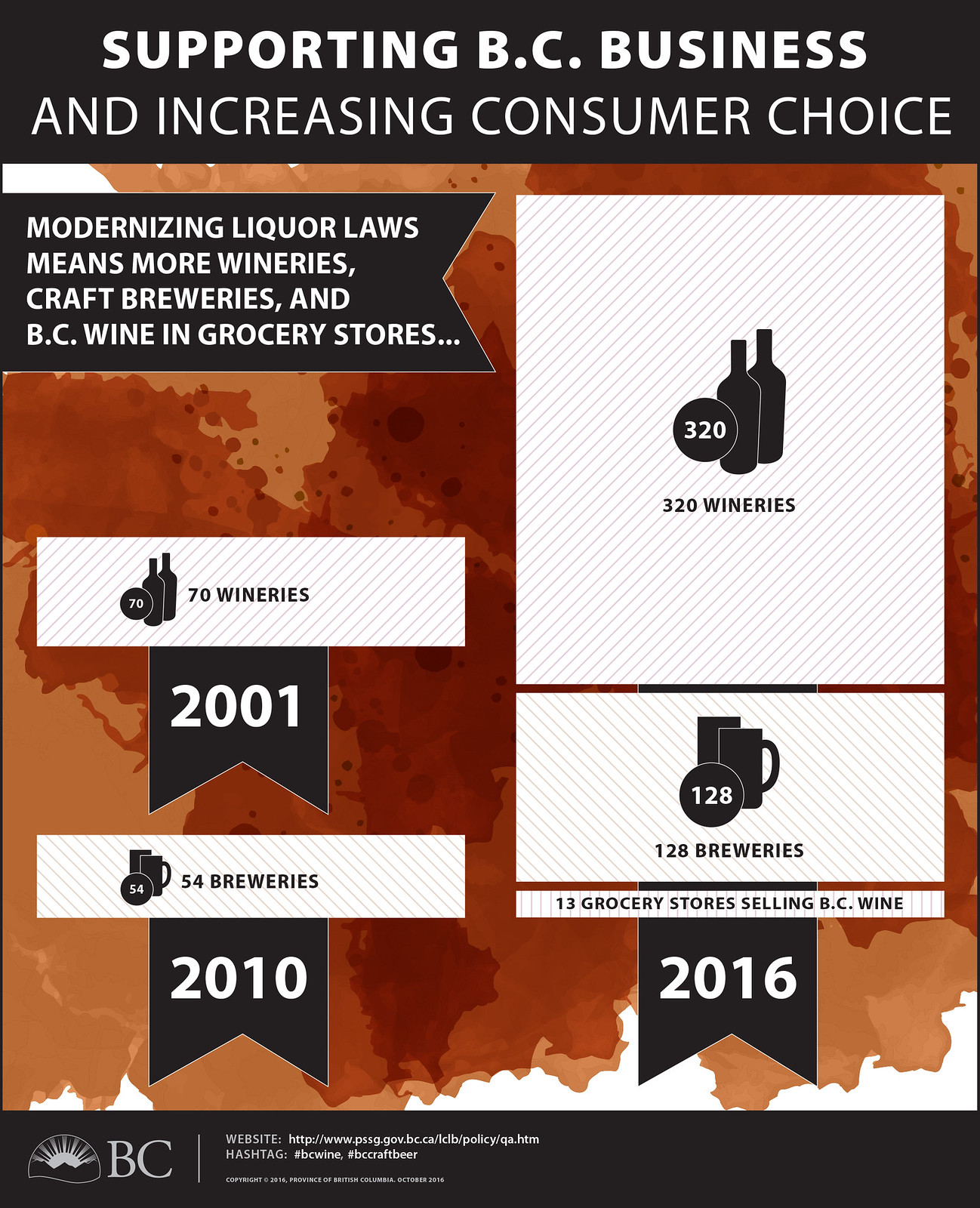The image features a visually striking graphic with a background in varying shades of beige, brown, and dark red, resembling tea or coffee stains. At the top, a black banner prominently displays the message, "Supporting BC business and increasing consumer choice." Directly below, another black area on the left reads, "Modernizing liquor laws means more wineries, craft breweries, and BC wine in grocery stores." 

The central part of the image is organized with white rectangular blocks containing silhouettes of wine bottles and beer mugs. On the left side, historical data is presented: a block showcases an image of wine bottles with the text "70 wineries" and "2001" in white on a black background, followed by another block showing beer mugs with "54 breweries" and "2010" similarly formatted. On the right side, updated figures for 2016 are depicted: two wine bottles are accompanied by "320 wineries," and beer mugs are paired with "128 breweries" along with "13 grocery stores selling BC wine."

At the bottom, a black border features the text "BC" followed by the website http://www.pssg.gov.bc.ca and hashtags such as #BCWine and #CraftBeer. Additional text and information appear, but are too small to be read clearly.